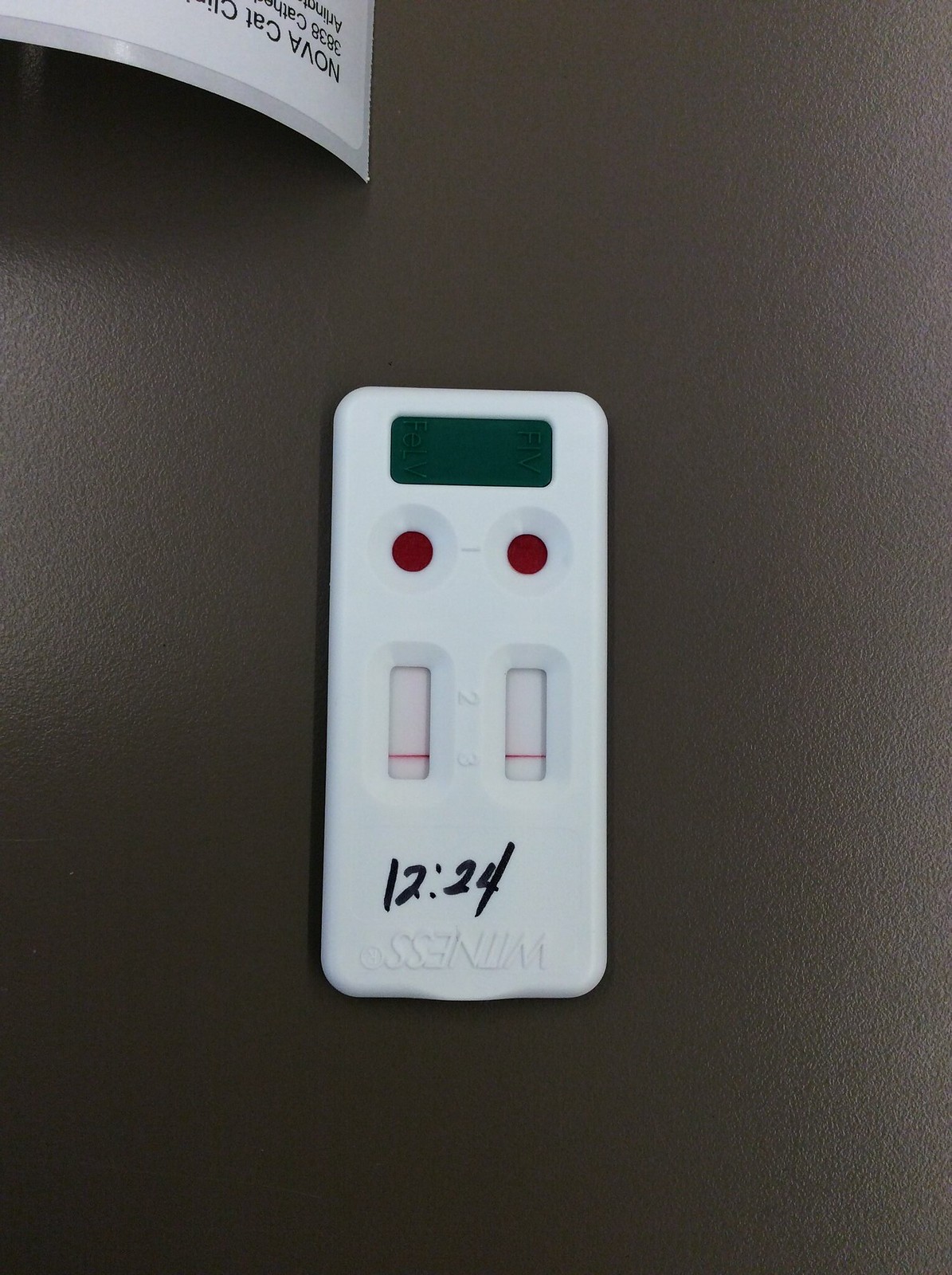In this rectangular photograph, there is a centrally placed rectangular white object against a dark brownish background. The background shades darker in the lower left corner and gets lighter toward the upper right, suggesting illumination from an overhead light source. The white object, which appears to be upside down, features several markings and elements.

At the bottom of this white object, the text "W-U-N-E-S-S" is partially discernible. Written in black marker, the numbers "12:24" are prominently placed, with a colon between "12" and "24." Above this, there is an open area resembling the reading window of a pregnancy test, with a single red line running horizontally across each of these rectangular sections. The digits "2" and "3" are also visible on the object.

Further up, there are two red circles of identical size positioned side by side. Above these circles, a small rectangular cut-out reveals the dark brown background underneath, adding depth to the composition. Overall, the image's intricate details provide a compelling focal point against the contrasting background.